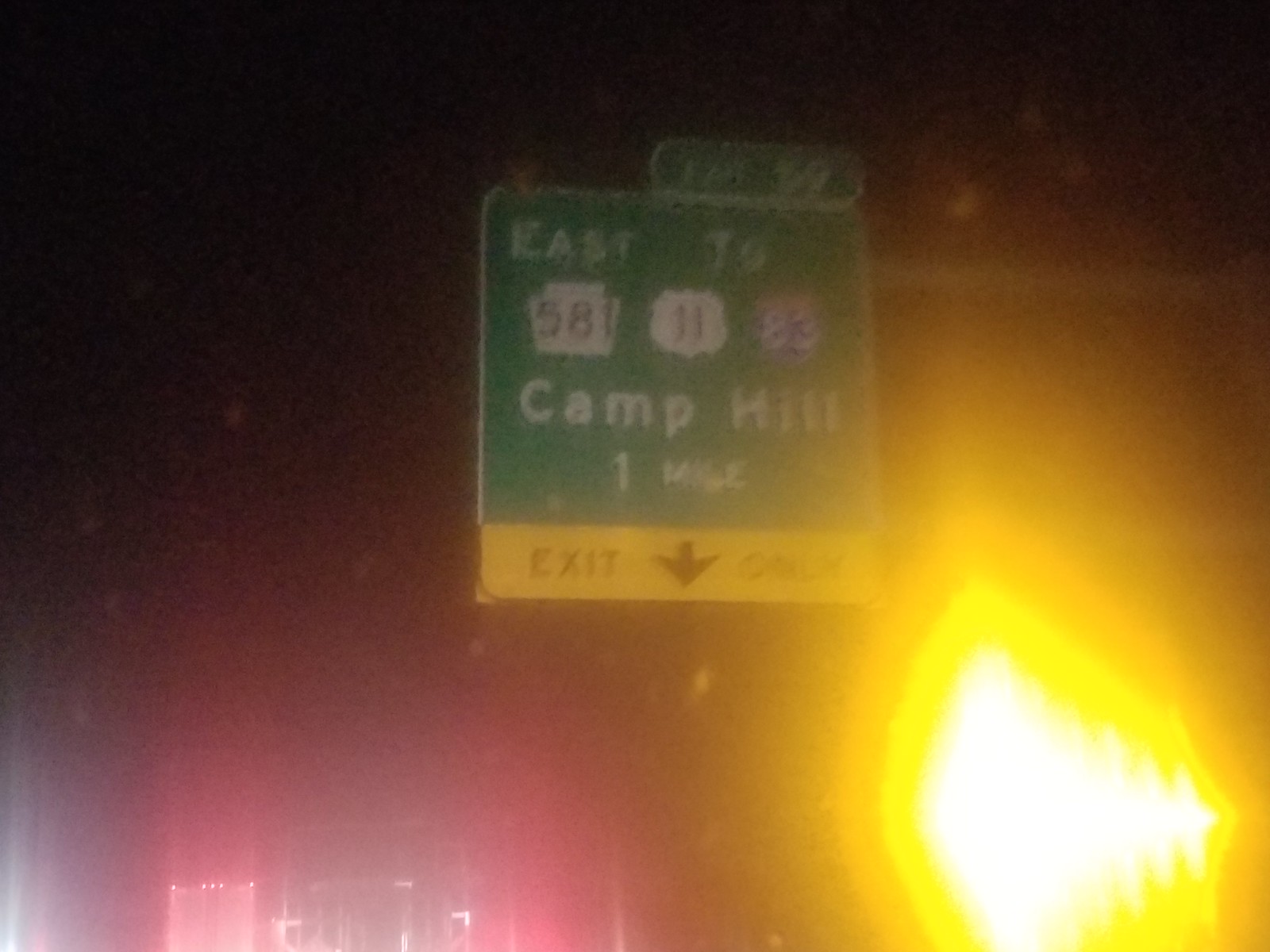The photograph captures a nighttime highway scene, slightly blurred and in low resolution. At the center of the image is a green highway sign with white lettering. The topmost part of the sign indicates "Exit 59," followed by "East." Below this, it references "58" in black lettering on a white background, and beside it, "11" within a white badge. Further to the right, another badge-like shape bordered in red and blue displays the number "83." Beneath these numbers, the sign directs towards "Uphill" and specifies "Camp Hill, One Mile, Exit Only" in a yellow banner with black letters, featuring a downward-pointing arrow. Additionally, the image captures a bright yellow light off to the right, possibly a vehicle blinker or a construction light. There's a visible pink lining to the left, likely from a truck, silhouetted against the dark, starless sky. The scene suggests the photo was taken from inside a moving vehicle, reflecting the blurry and distorted effects of motion and artificial lights.